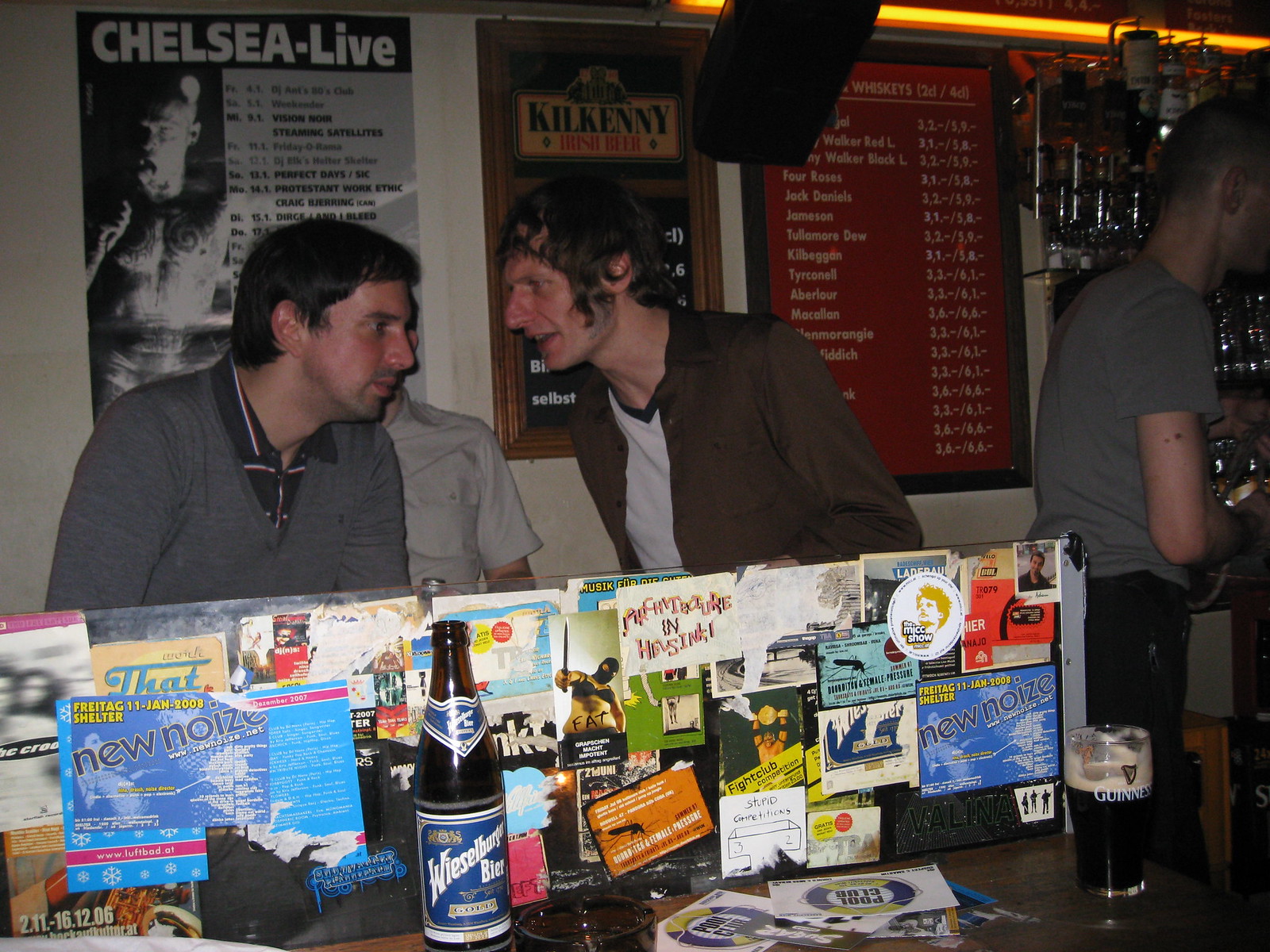In a color photograph taken inside a pub, four men are depicted behind a table cluttered with multiple concert flyers. At the forefront, a large bottle of "Weissmurger Beer" and a clear glass labeled "Guinness," three-quarters full of dark beer topped with froth, are placed. Two central figures are engaged in conversation: the man on the left sports a gray shirt over a blue undershirt, revealing a blue collar at his neck, and has black hair with some redness on his Caucasian face. The man to his right, distinguishable by his messy brown hair and a red-tinged face, wears a brown jacket over a white shirt. Behind them, a third man’s face is partially obscured, identifiable only by his gray short-sleeved t-shirt and black pants. Far right, a thin man with short hair stands with his back to the camera, more of the pub's ambiance in view—various signs advertising music events and beers, including a red sign with names and scores, and a poster titled "Chelsea Live" featuring a monochrome image of someone holding an item in their mouth. The wall behind the central figures is adorned with cards, pictures, and clippings, adding to the lively atmosphere typical of a bustling bar.